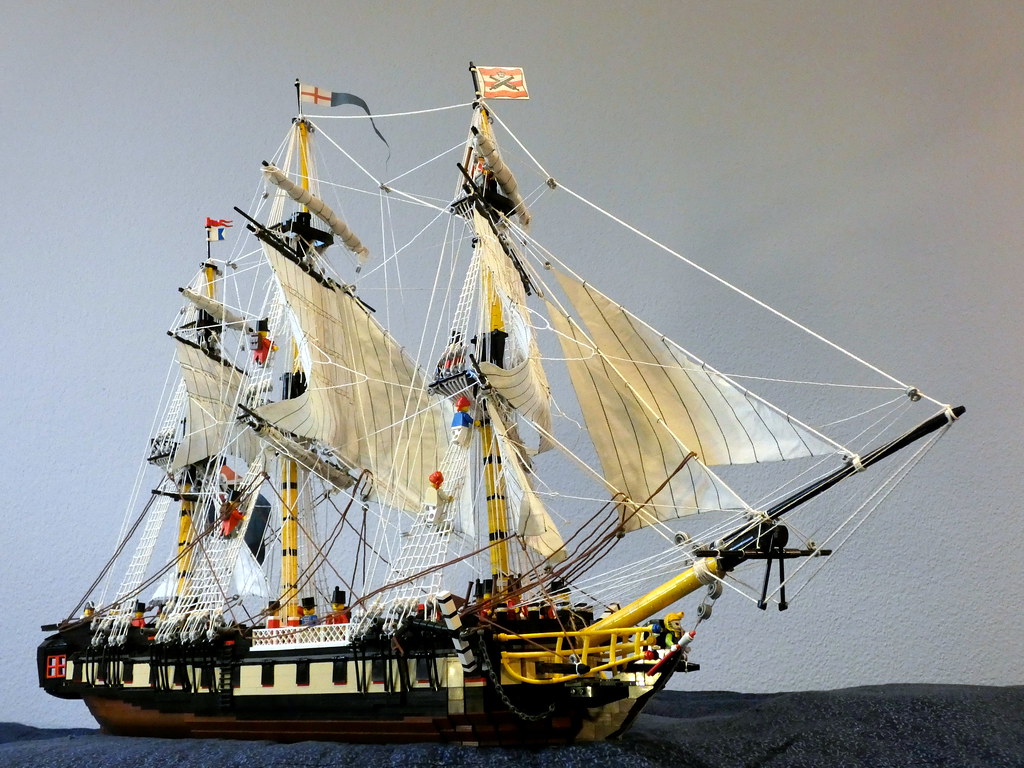The image displays an intricately crafted Lego model of an ancient sailing ship set against a backdrop that appears to be a light gray painting on a wall. The sea is represented by a dark blue, possibly bluish gray, blanket or fabric. The ship itself is predominantly black, white, brown, and yellow, with additional accents of red and blue. The model features fabric sails—white with black stripes—supported by seven masts, each adorned with flags. At the top, there's a red and white striped flag marked by a blue or black X, alongside a flag with a red cross on a white field and another flag displaying crossed cannons. Scattered throughout the ship, from bow to stern, are numerous Lego figurines, with some even climbing the nets to the sails. The overall scene, captured in what seems to be a casual, non-professional photograph possibly sourced from a social media page, is both detailed and immersive, highlighting the layered construction and variety of materials used in the model.